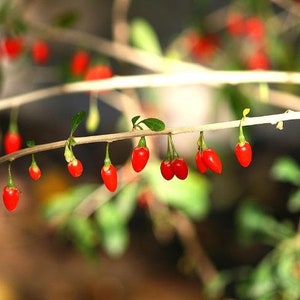In this close-up, daytime photograph taken outside on a sunny day, a light brown branch is prominently displayed at the center of the composition. The branch is adorned with strikingly bright red fruits, each resembling tiny bell peppers or Christmas lights due to their vivid coloration and bulbous shape. These small fruits are attached to the branch by lighter green stems and are occasionally paired but mostly hang singly. Surrounding the central branch, several other branches appear in the background, similarly bedecked with the same red fruits. The blurred backdrop reveals a variety of leaves, trees, and bushes, hinting at a lush garden setting. The ground beneath the branches is dusky, possibly covered with grass or brown dirt, enhancing the contrast with the vibrant fruits. The sunlight bathes the entire scene, emphasizing the colors and creating a lively natural tableau.